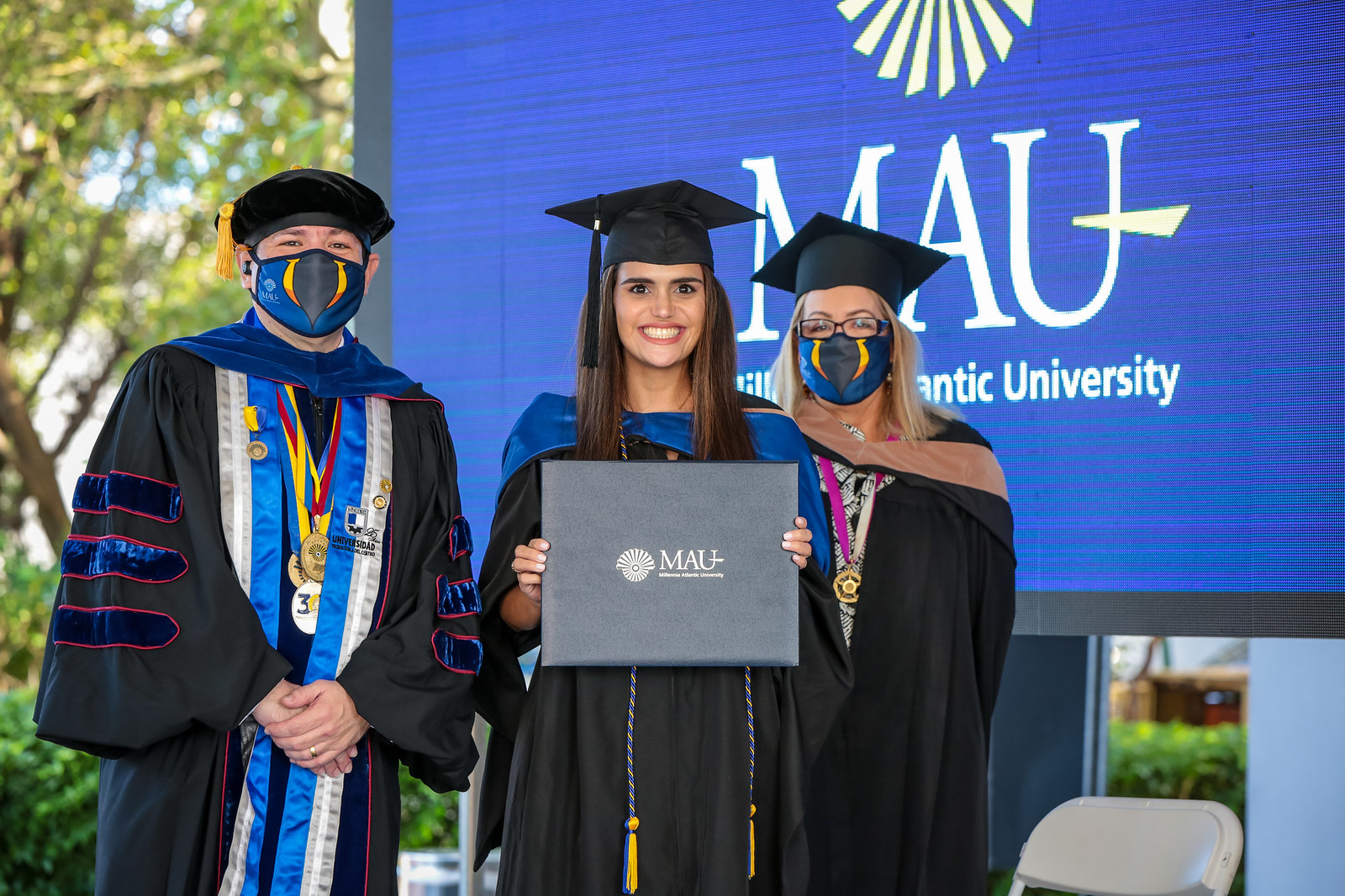In the photo, three individuals are celebrating at what appears to be a university graduation ceremony outdoors, framed by a natural backdrop of trees. Dominating the right side of the image is a large screen displaying the blue and white logo of Millennia Atlantic University (MAU), though part of the text is cut off. The trio stands proudly before the screen.

On the left is a man dressed in a black graduation cap with a gold tassel, wearing a face mask and layered in multiple medals over his black robe adorned with white and blue accents. He exudes an air of accomplishment. At the center is a young woman, beaming widely, with long brunette hair cascading below her black graduation cap. She holds a booklet likely containing her degree, featuring the MAU logo, and wears a blue shawl draped over her black graduation robes. To her right is an older woman with long blonde hair, also in graduation attire, including a black hat, a brown and black shawl, and a mask. She wears glasses and dons two medals around her neck, signifying her achievements.

The group encapsulates the triumph and joy of graduation day, unified by their MAU regalia and the celebratory mood of the occasion.